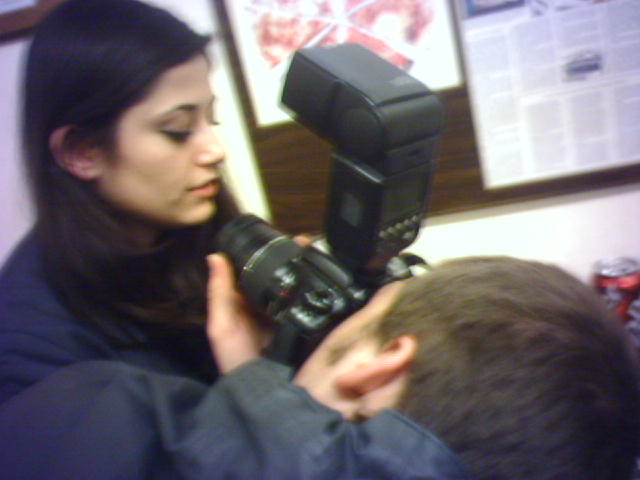In this blurry and out-of-focus interior photograph, a young man in a blue jacket with a hood down is captured leaning slightly to the right as he concentrates through the viewfinder of a large DSLR camera. The camera, equipped with a tall tower flash, is directed towards a young Latina woman with dark brown hair, who appears to be looking down, possibly at a table, document, or the floor. The setting features white walls illuminated by artificial lighting, and in the background, there's a brown wood bulletin board adorned with multiple posters, including one depicting pizza on a white background and another covered with small black fonts. The unclear details due to the blurriness add a sense of distortion to the scene, making it more challenging to discern the finer elements.